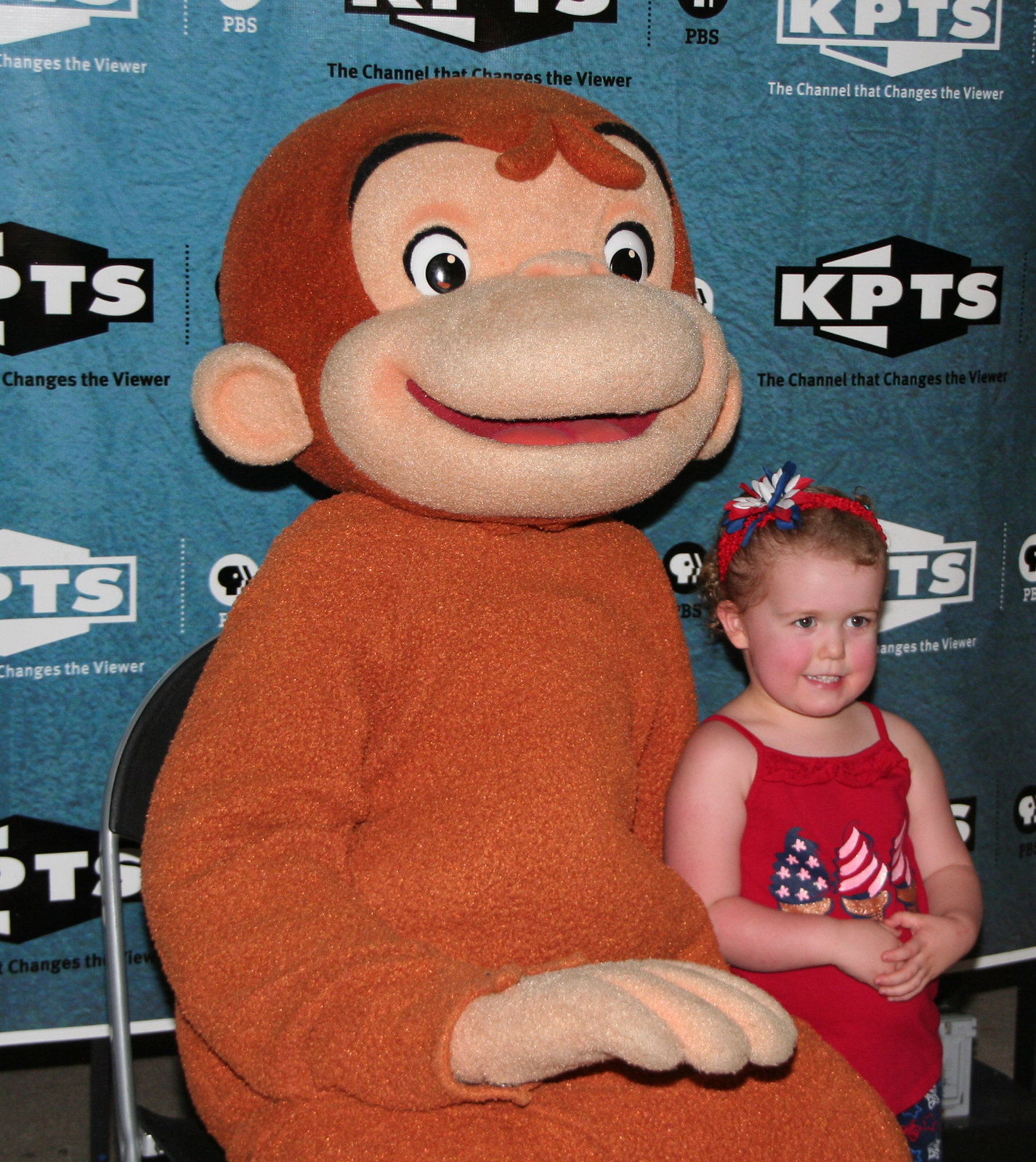In the image, there is a young girl, about one or two years old, standing in front of a light blue backdrop adorned with KPTS logos in alternating white and black lettering. The KPTS logos are on a repeating pattern covering the entire background. The little girl is wearing a vibrant red sleeveless dress featuring illustrations of three colorful sailboats, with one sporting a blue sail, another with a striped sail, and the third sail's color not clearly visible. She has a red, white, and blue ribbon in her hair and is standing with her hands clasped in front of her. To her right, there is a large stuffed mascot resembling Curious George. The mascot has a darker brown head with beige facial features and a lighter brown body. This charming scene seems to be captured at a photo opportunity, possibly during an event celebrating an American holiday like the 4th of July.